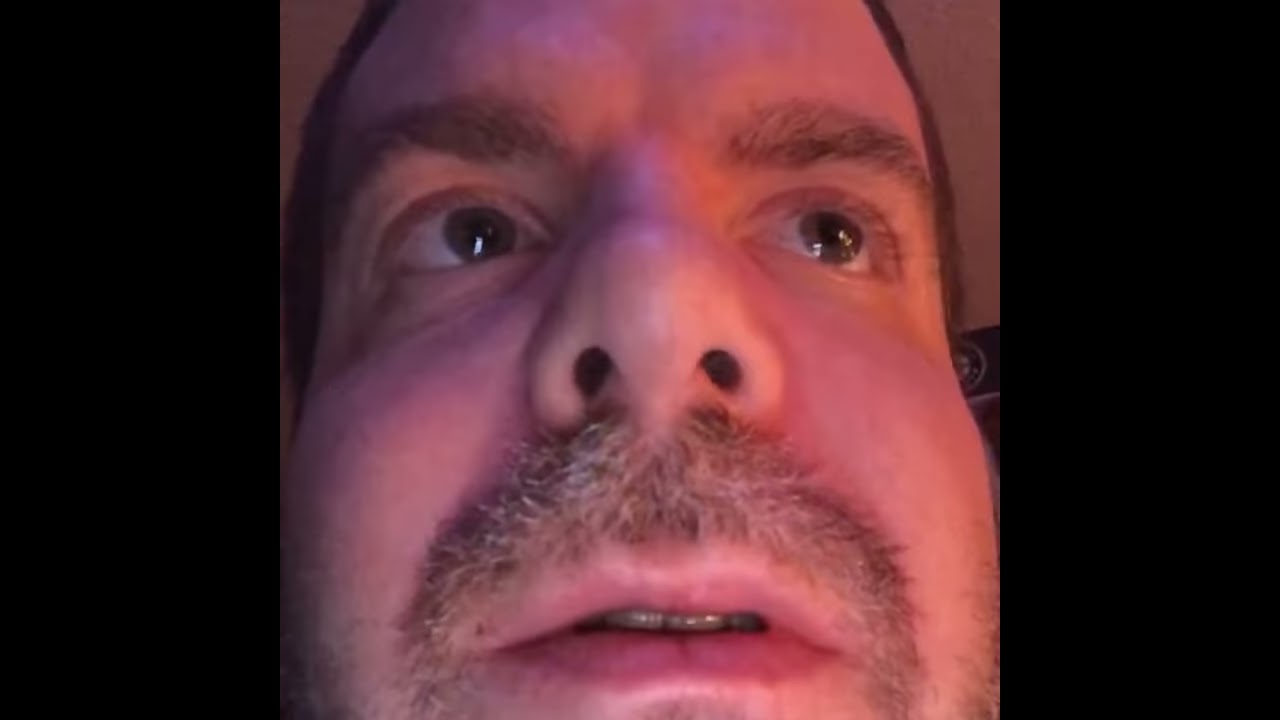This highly detailed close-up image captures an expressive segment of an older Caucasian man's face, zoomed in from just above his chin to almost the top of his forehead. His prominent gray and brown mustache, speckled with white hairs, accentuates the area beneath his nose. The man's mouth is partially open, revealing his two large, front buck teeth. His thin lips have a subtle red hue. His gray eyes, which reflect three light sources, are directed upwards and to the left, suggesting he is observing something in the distance. His brown, arched eyebrows and the visible strands of brown hair indicate a thinning, balding scalp. The background shows a white-colored ceiling with a logo on the wall, slightly to the right. Dark vertical bars frame the image on both sides, emphasizing the intense focus on the man's facial features.